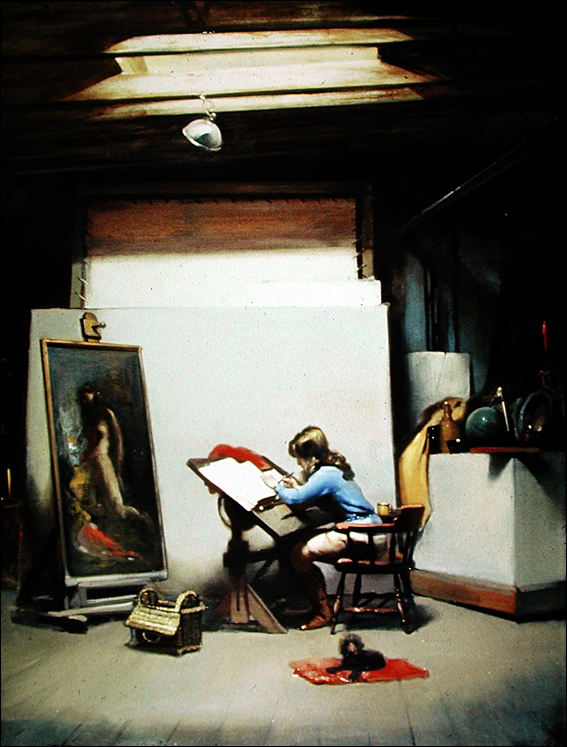In this detailed and captivating painting, a young woman artist is depicted in her studio, deeply engrossed in her work. She sits on a wooden chair, leaning over an inclined desk reminiscent of those found in historic scriptoria. Clad in a blue shirt and tan pants, her left hand rests on a large book while her right hand actively writes or draws within it. The studio environment is rich with creativity, featuring a series of tall, blank canvases standing in the background and a completed painting of a human figure to her left. A large, vertical painting positioned to her left also catches the eye – possibly the reference for her current work. The lighting is a significant feature, with a lantern-like fixture hanging from the ceiling amidst exposed rafters, illuminating the scene with warm hues of orange, red, brown, beige, yellow, blue, white, gray, tan, and black. On the floor near her, a small dog sits attentively on a red blanket, adding a touch of warmth and companionship to the scene. Further enhancing the cozy atmosphere, a basket is positioned on the floor to her left, and a variety of indistinct items adorn a desk behind her. The painting radiates an old-fashioned charm, reminiscent of Norman Rockwell's style, combining meticulous detail with a narrative quality that invites viewers into the artist's world.